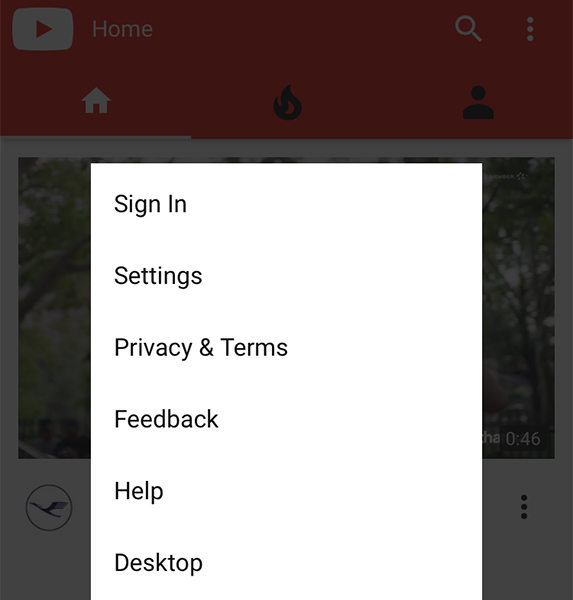The image features a vibrant red background with a variety of elements arranged across it. At the top left, there is a small white square and a play button icon. Adjacent to these are icons for home, a magnifying glass for search, and a menu represented by three dots (...).

Central to the image, a section with a white background draws the eye, housing options such as "Sign In," "Settings," "Privacy and Terms," "Feedback," "Help," and "Desktop." 

In the background, lush green foliage is noticeable, adding a natural touch to the scene. At the bottom right corner, the number "046" is visible, along with another set of three dots (...). Towards the bottom left, an image of a bird stands out alongside the YouTube logo and additional text related to YouTube settings.

Prominently, a house and the depiction of fire are also part of the scene, contributing to the overall eclectic and detailed composition.